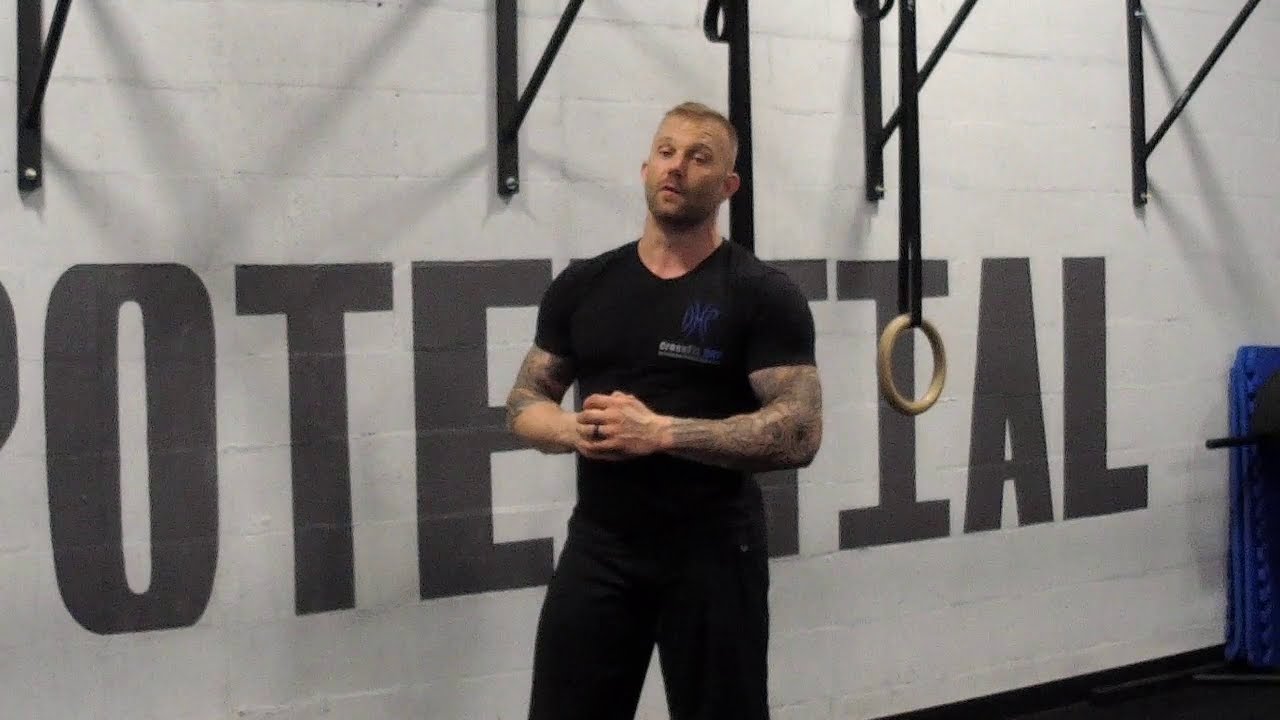The photograph captures a muscular, white male trainer, possibly in his mid-30s to early 40s, positioned centrally within a gym setting. He has short hair and a closely trimmed beard, with tattoos adorning both his arms. He is donned in a fitted black t-shirt, featuring an unreadable logo, and black pants. The man stands with his hands clenched together in front of him, body angled slightly to the left, and his gaze directed off to the left side of the viewer. Dominating the backdrop is a white cement brick wall, partially obscured by the man, with black capital letters that spell out "POTENTIAL." Adjacent to him, on the right, is a gymnastic ring, reinforcing the CrossFit gym ambiance suggested by the surroundings and equipment.